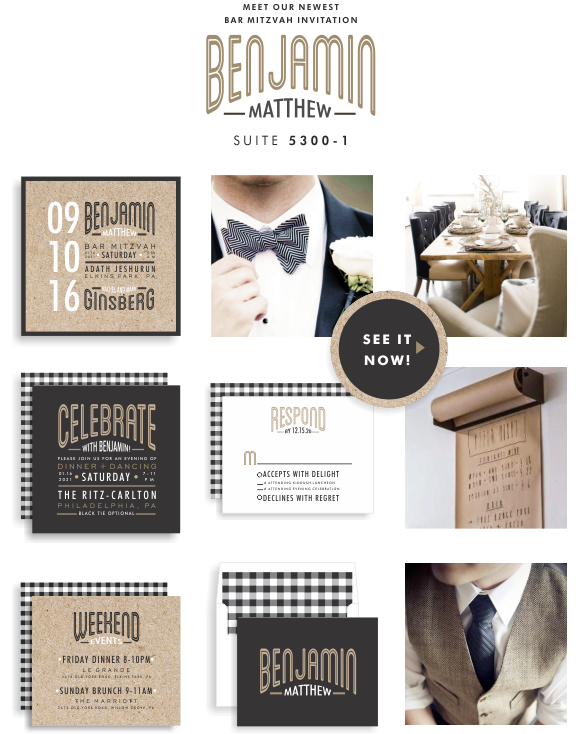The image is a detailed digital brochure for the Bar Mitzvah of Benjamin Matthew, scheduled for September 10, 2016. At the top, text reads "Meet Our Newest Bar Mitzvah Invitation, Benjamin Matthew, Suite 5300-1." The layout consists of nine distinct images arranged in three columns. 

**Left Column:**
1. The date "9-10-16" along with the text "Benjamin Matthew, Bar Mitzvah Saturday, Adam Jeschron, Ginsberg."
2. An invitation to "Celebrate with Benjamin: Dinner, dancing, Saturday at the Ritz Carlton, Philadelphia PA, black tie optional."
3. A schedule of weekend events: "Friday dinner from 8-10 pm, Saturday brunch from 9-11 am."

**Middle Column:**
1. A close-up image of a young man wearing a dark blue jacket, a white shirt, and a striped bow tie with a carnation on his lapel.
2. An RSVP card with the options to "Accept with delight" and a call to respond.
3. An envelope with a plaid interior and a card that reads "Benjamin Matthew."

**Right Column:**
1. A long, elegantly set dining table with black chairs on the sides and a beige chair at the end.
2. A scroll of brown paper with Hebrew writing or a printed schedule.
3. An image of a young man in a white shirt, a blue tie, and a light brown vest.

This brochure elegantly mixes formal announcements with intimate visual details, perfectly capturing the spirit of Benjamin Matthew's upcoming celebration.